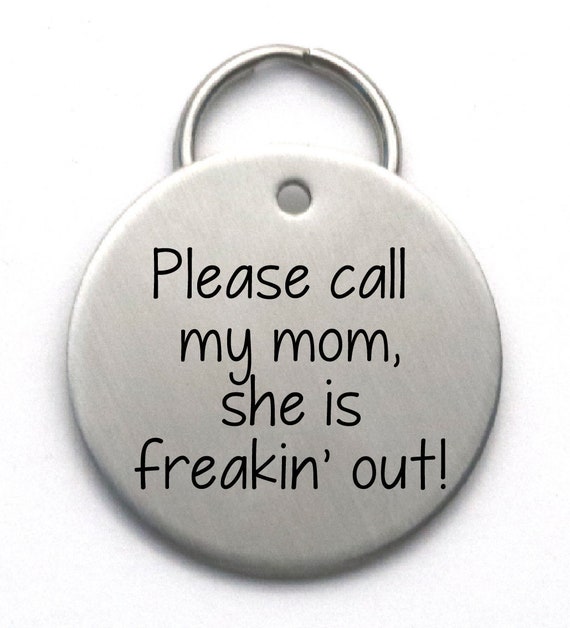The image features a computer-generated clipart of a round, silver dog ID tag. The tag, resembling brushed aluminum, has a small hole at the top with a key ring attached, allowing it to connect to a dog collar. The circle is beveled, with a highlighted top left side and a darker, shaded bottom right. Centered on the tag is black text that reads: "Please call my mom, she is freakin’ out," with "freakin’" spelled F-R-E-A-K-I-N apostrophe. The message appears clearly written and looks like it was typed on a computer. The white background ensures that the focus remains solely on the tag, which looks like it could be used as a novelty item or as an additional piece of identification on a pet's collar.